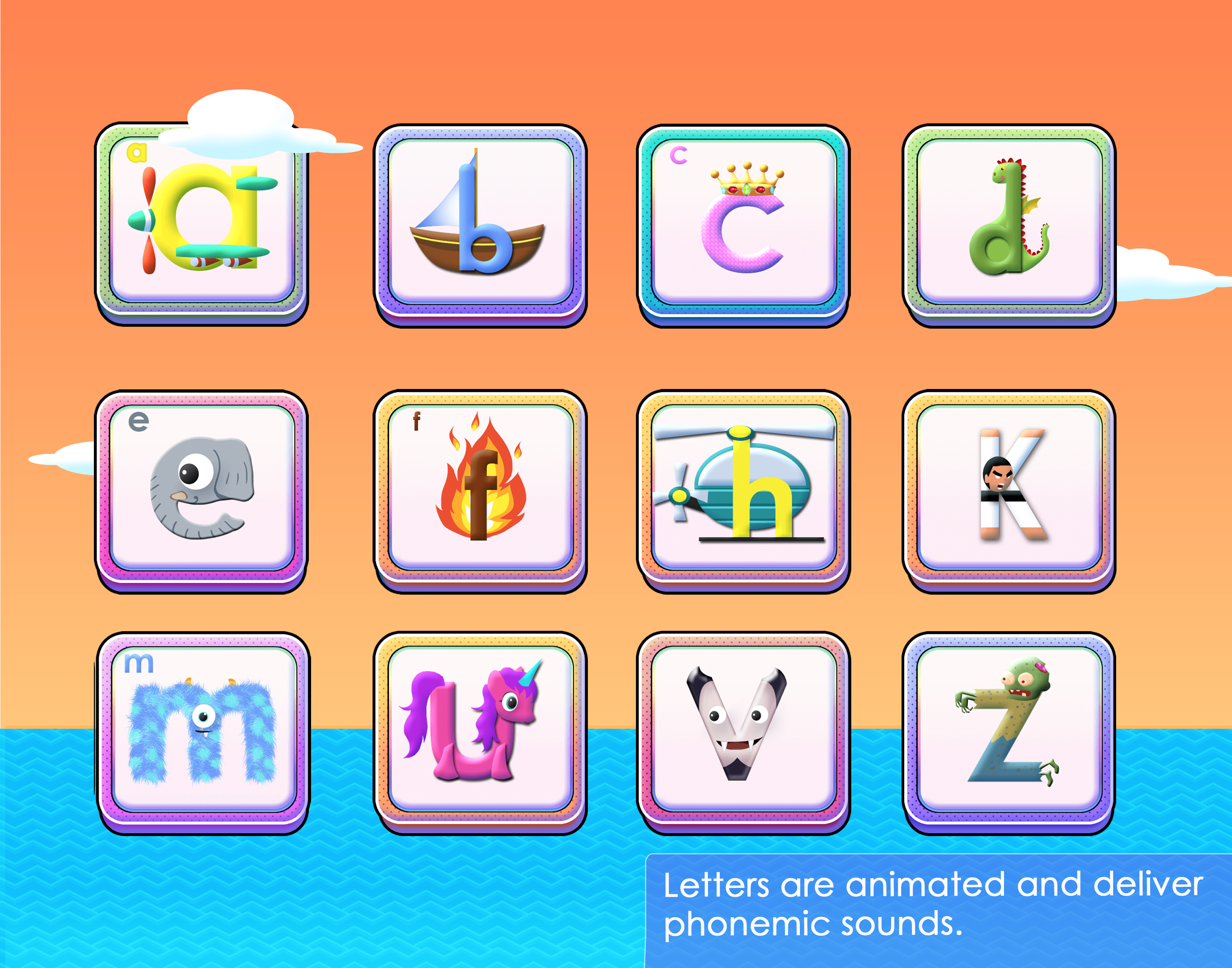This vibrant, educational image is divided into two distinct sections. The top half features a playful orange sky adorned with fluffy white clouds, while the bottom half depicts a serene blue ocean with stylized waves drawn in straight lines. In the bottom right corner, the background shifts to a deeper blue with white text that reads, "Letters are animated and deliver phonemic sound."

At the center of the image, there are twelve colorful squares with rounded corners, each showcasing a specific letter paired with an animated illustration. These squares are organized in a structured layout: four in the top row, four in the middle row, and four in the bottom row, though the bottom row extends slightly to the right.

1. **A (Top left)**: A yellow letter 'A' accompanied by an animated aeroplane soaring through the sky.
2. **B**: A blue letter 'B' with a brown boat gently floating on water.
3. **C**: A purple letter 'C' crowned by a regal yellow crown.
4. **D (Top right)**: A green letter 'D' next to a friendly green dinosaur.
5. **E (Middle left)**: A letter 'E' depicted with a gray elephant.
6. **F**: A letter 'F' ignited by yellow flames.
7. **H**: A letter 'H' flying alongside a helicopter.
8. **K**: A letter 'K' with its corresponding image (not specified, but implied by the pattern).
9. **M**: A letter 'M' with a quirky monster.
10. **U**: A purple letter 'U' paired with a magical unicorn.
11. **V**: A letter 'V' illustrated with a black and white vampire.
12. **Z**: A letter 'Z' with a zombie colored in green and blue.

Each animated letter is designed to help children recognize phonemic sounds while engaging with colorful and imaginative visuals.